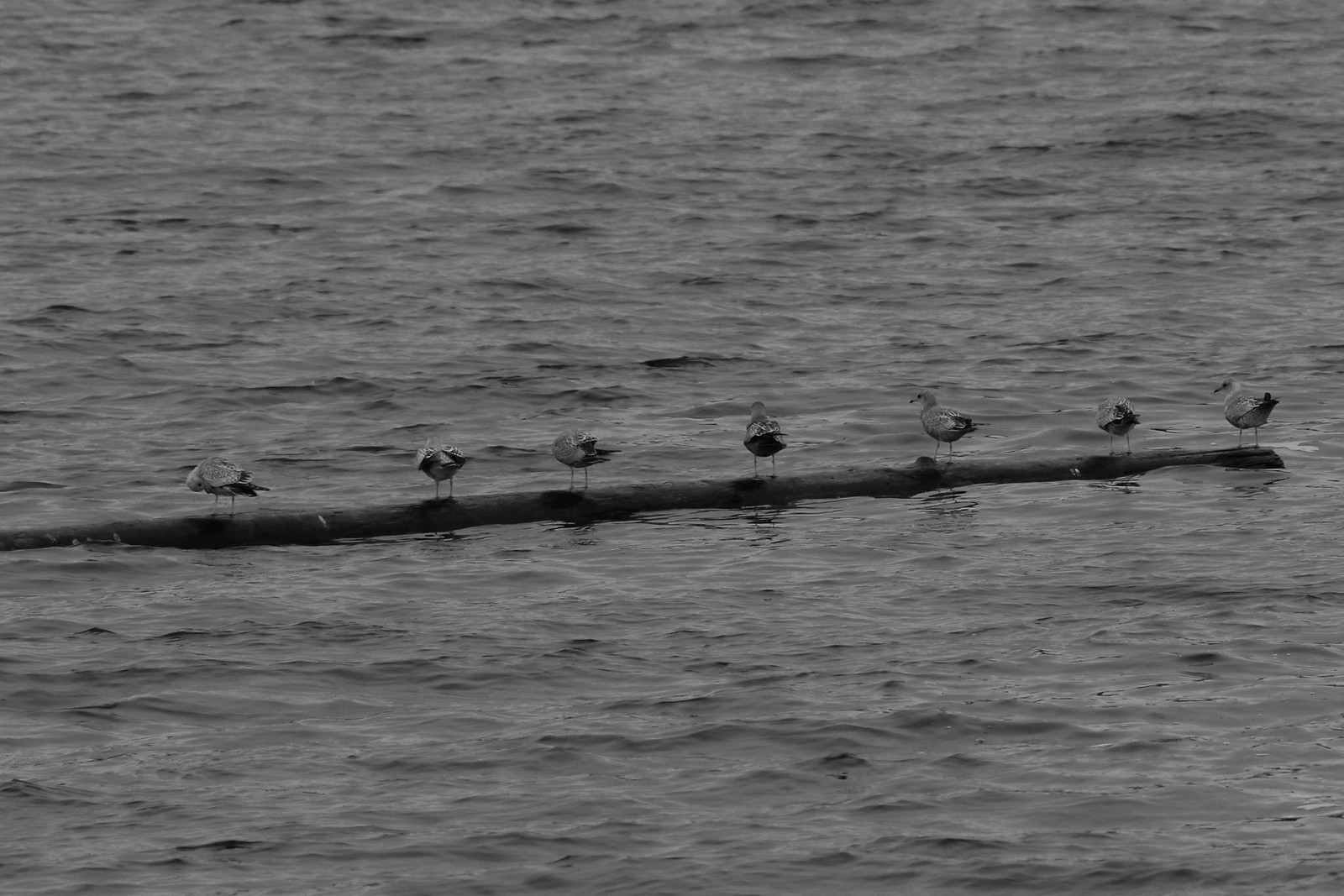This black-and-white photograph features seven seagulls standing in a line on a slim, floating log in a serene body of water. The water's surface is calm, with gentle waves softly rippling. The seagulls, varying in shades of gray, are all facing the same direction towards the left, displaying their backsides and long, skinny legs. The third bird from the left is preening itself, while the fifth bird appears to be looking at its left-hand neighbor. The log, resembling a thin sapling, is the sole structure visible against the placid aquatic backdrop, suggesting the setting might be a tranquil lake. The photograph captures a quiet, still moment without any other objects, people, or landscape elements in view.